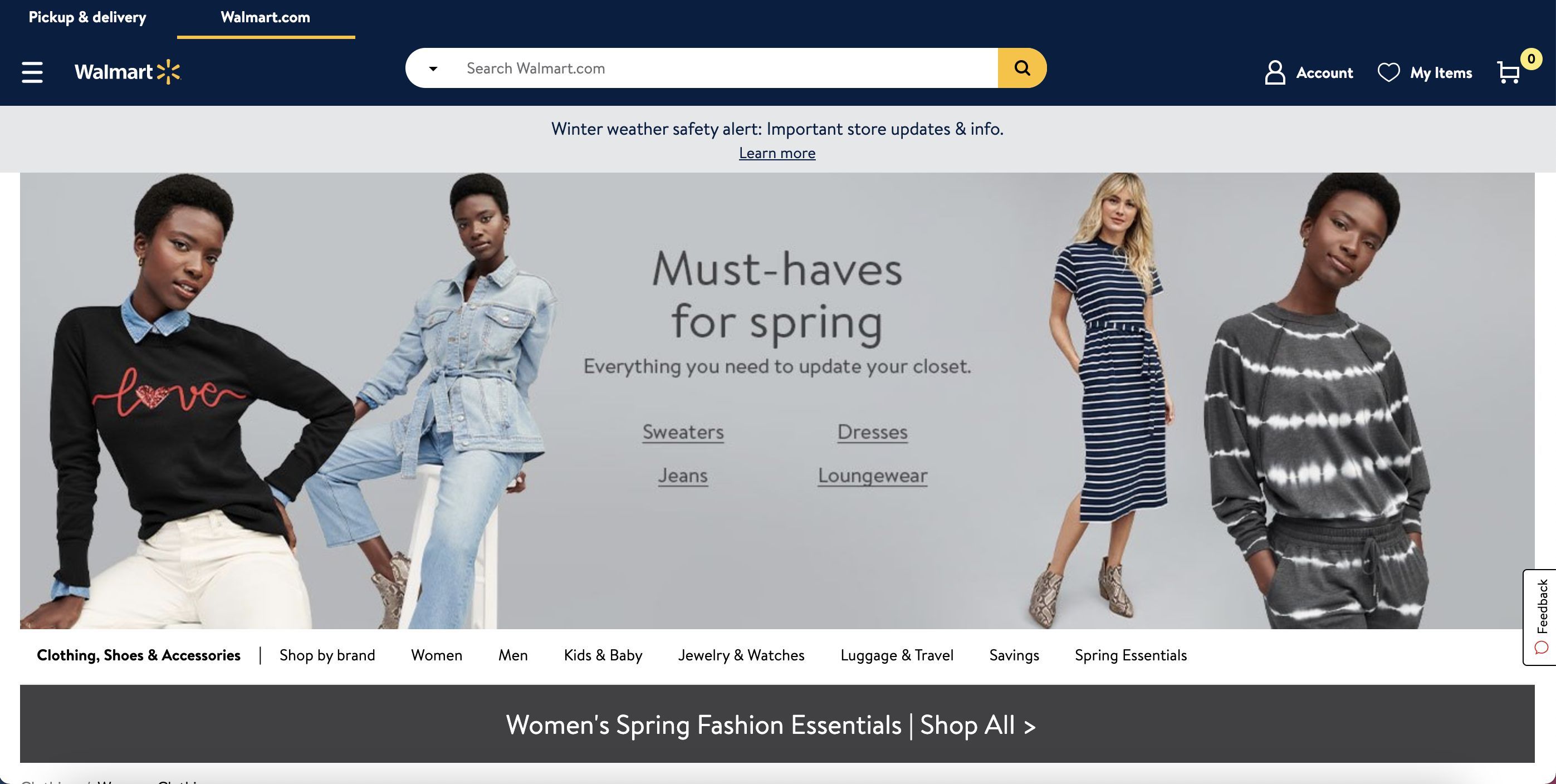This screenshot showcases the Walmart webpage, characterized by its distinct blue banner at the top. On the left corner of the banner, small white text reads "Pickup & Delivery," followed by "walmart.com." A yellow line runs beneath "walmart.com." Positioned to the left below this line, there is a three-line icon beside the Walmart logo. Centralized in the banner is a search bar that prompts "Search walmart.com" in small black letters, flanked by a drop-down box on the left and a magnifying glass icon with a yellow background on the right. To the right side of the banner, the options "Account," "My Items," and a shopping cart icon are displayed.

The main body of the page begins with a gray border at the top, featuring a prominent winter weather safety alert, including important store updates and information, all written in blue letters. This notice invites users to "Learn More."

Below the alert, a large promotional image features four women—two on the left and two on the right—modeling various outfits. Centered in this image, a bold text announces "Must-haves for Spring: Everything you need to update your closet." Beneath, categories such as "Sweaters," "Jeans," "Dresses," and "Loungewear" are listed as hyperlinks.

At the bottom of the screen, a gray banner highlights "Women's Spring Fashion Essentials" with a "Shop All" option, all centered in white text.